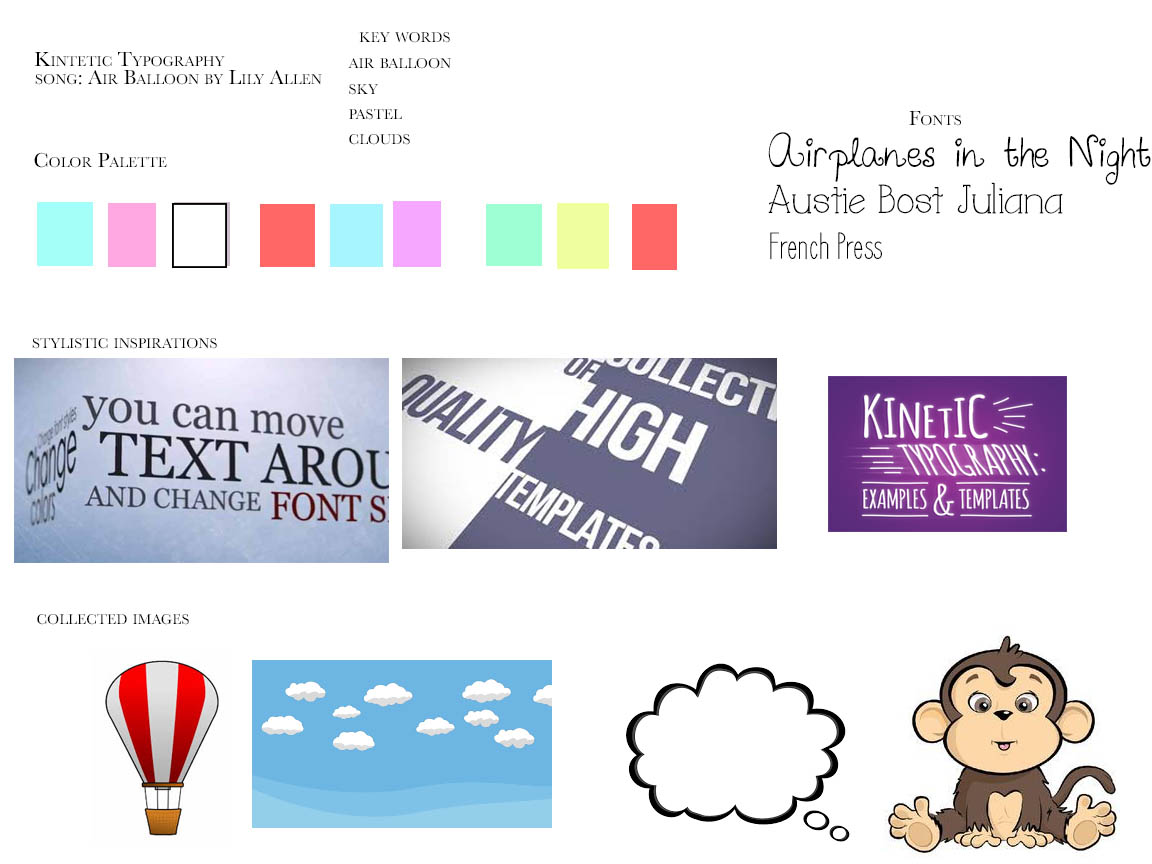The image is a detailed web page for kinetic typography design inspired by the song "Air Balloon" by Lily Allen. In the top left corner, it features the title "Kinetic Typography" incorrectly spelled as K-I-N-T-E-T-I-C. Below, it lists the keywords: Air Balloon, Sky, Pastel, and Clouds. The page displays a pastel color palette with various shades of pink, teal, yellow, and red. To the right, it presents a selection of fonts: Airplanes in the Night, Austie*, Boast, Juliana, and French Press, each showcased in its respective style. Beneath the fonts, the section titled "Stylistic Inspirations" exhibits several text backgrounds with different design ideas. At the bottom, "Collected Images" includes a series of cartoon-like drawings: a red-and-white striped hot air balloon, a blue sky with puffy white clouds, a thought bubble, and a baby monkey. The overall aesthetic suggests that these elements might be part of a broader brand marketing package or design template collection, although its exact purpose remains somewhat unclear.